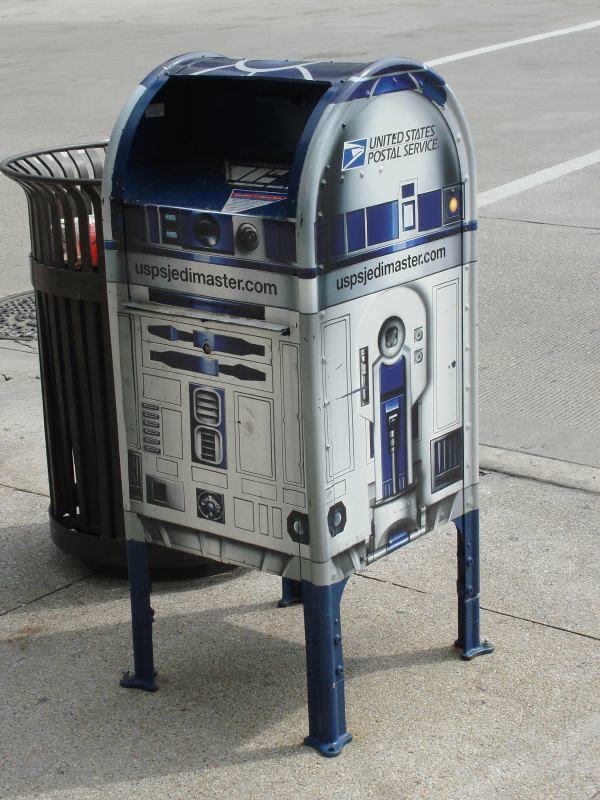The image features a city mailbox on a sidewalk, creatively designed to replicate R2-D2 from Star Wars. The mailbox is predominantly white and blue, with intricate details mimicking R2-D2's body, including dials, lights, and leg-like structures at the base which are dark blue. The upper part of the mailbox is blue, while the central body area is silver and bears the website "USPSJediMaster.com" in black text, both on the front and the right side. Additionally, the right side of the mailbox displays the United States Postal Service name and its emblem, the blue and white eagle head. Adjacent to the mailbox is a black metal garbage can and a gray manhole cover is visible in the road nearby. The background reveals a street with visible stripes and a crosswalk leading across it.